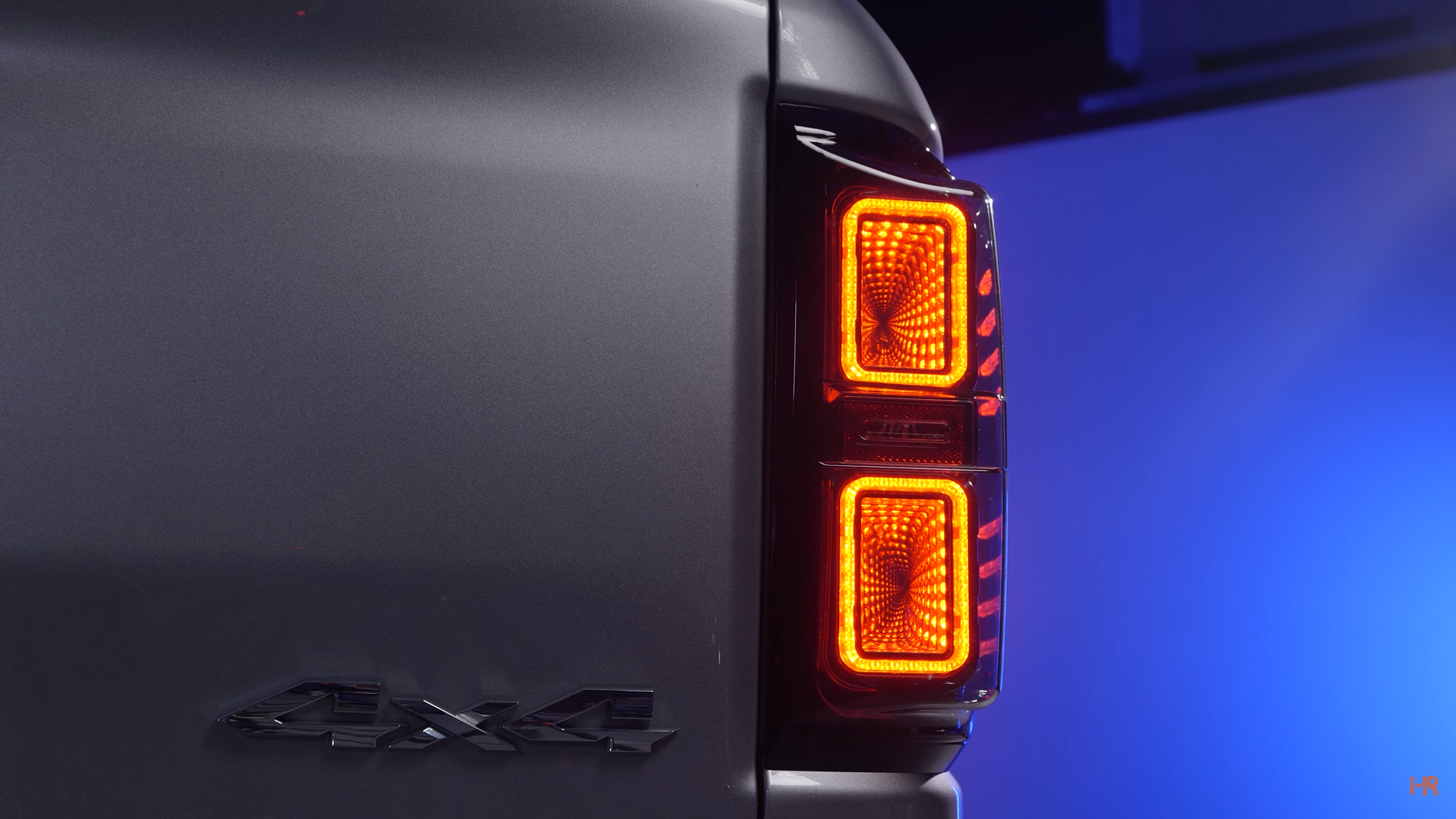This image is a detailed, 3D color illustration in landscape orientation, focusing on the back of a gray 4x4 vehicle. The primary subject is the right rear taillight, which is vertical and centrally positioned in the image. The taillight has a black plastic casing with a slanted top, and features stacked, rectangular lights with rounded corners. These lights emit a yellow to yellow-orange gradient and are lit, bordered by the black casing. Additionally, we see some red lights on the side of the case. On the bottom left of the vehicle's body, there's a chrome decal reading "4x4." The background of the illustration is a vivid blue wall, with a smaller blue item visible at the top. In the bottom right corner, the letters "HR" appear in orange.